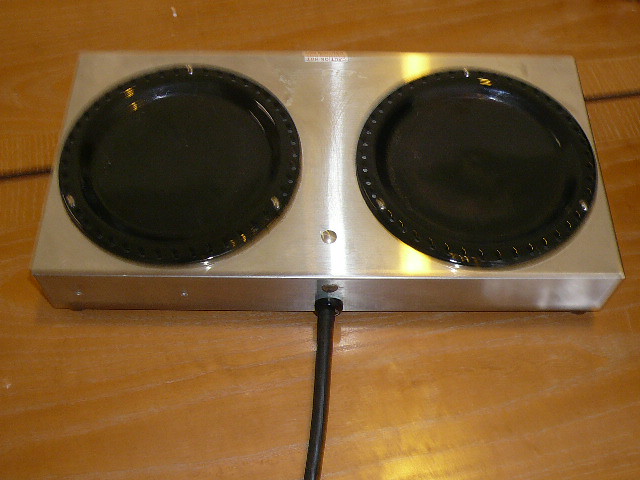The rectangular photograph, taken indoors, gives a top-down view of a light brown wooden surface, which appears slightly yellow in certain areas due to light glare from above. The wood grain runs horizontally from left to right. Situated on this surface is a rectangular, silver metal box with a black cord extending from the bottom center of the photo to the midline, where it connects to the box. On top of the box are two equally sized, round black plates, one on the left and one on the right, resembling heating elements often found in portable stoves or warming plates for coffee pots. The stainless steel box, reflecting yellow and white light, has a small rectangular white sticker with black, blurry, and partially upside-down text that includes the word "hot.” The entire setup rests on the wooden table, emphasizing the device’s function as a heating apparatus.